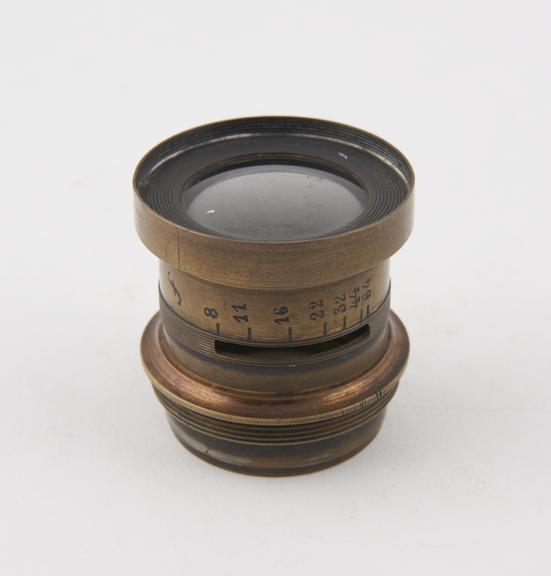The image showcases an antique camera or telescope lens positioned upright on a pristine white background, devoid of any surrounding objects. The lens features a rustic, cylindrical body with a bronze or copper finish, exhibiting a touch of patina that subtly enhances its vintage charm. At the top, a glass lens is encased by a blackened ring, hinting at age and usage. Numbered markings — 8, 11, 16, 22, 32, 44, and 64 — run down the side of the lens, likely indicating aperture settings, accompanied by a stylized "F" just above them. The overall structure includes screws and threading, suggesting it can be mounted or adjusted, with some parts extruded from the main cylinder.